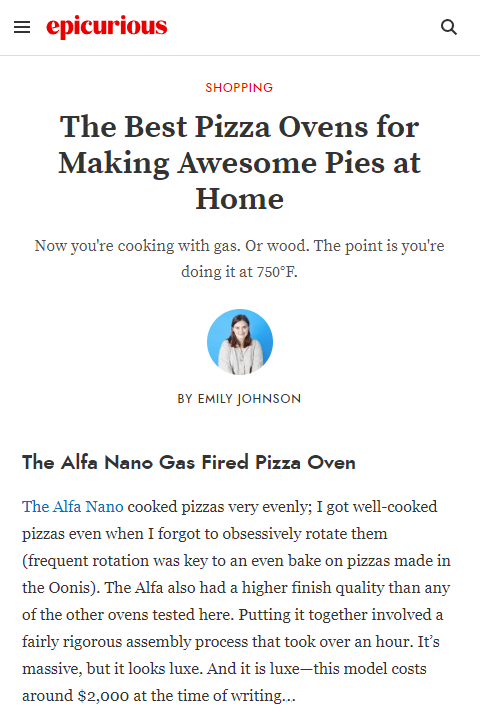This image showcases an article from the Epicurious website, viewed on a mobile device in landscape mode, which gives the display a very narrow appearance. The background of the site is white, contributing to a clean and organized look. 

**Layout:**
- **Top Left Corner (Navigation):**
  - Black menu icon.
  - To its right, the iconic Epicurious logo is prominently displayed in red.
  - Far right, there's a black search icon.
  
- **Main Heading:**
  - Centered at the top, "SHOPPING" is highlighted in bold, capital red letters.
  - Directly below, the main article title "The Best Pizza Ovens for Making Awesome Pies at Home" is presented in large, bold, black letters.
  
- **Subtitle:**
  - Below the main title, a descriptive subtitle reads, "Now you're cooking with gas or wood. The point is you're doing it at 750 degrees Fahrenheit," in small gray letters.
  
- **Author Information:**
  - Below the subtitle, centered, is a small circular profile photo of the author.
  - Under the photo, the author's name "BY EMILY JOHNSON" is displayed in capital gray letters.
  
- **Article Content:**
  - Sub-heading on the left: "The Alfa Nano Gas Fired Pizza Oven" in large black letters.
  - Beneath this sub-heading, a detailed description of the experience with the Alfa Nano Gas Fired Pizza Oven is provided.

The structured layout and concise headings highlight crucial elements, making it easy for readers to navigate through the content seamlessly.